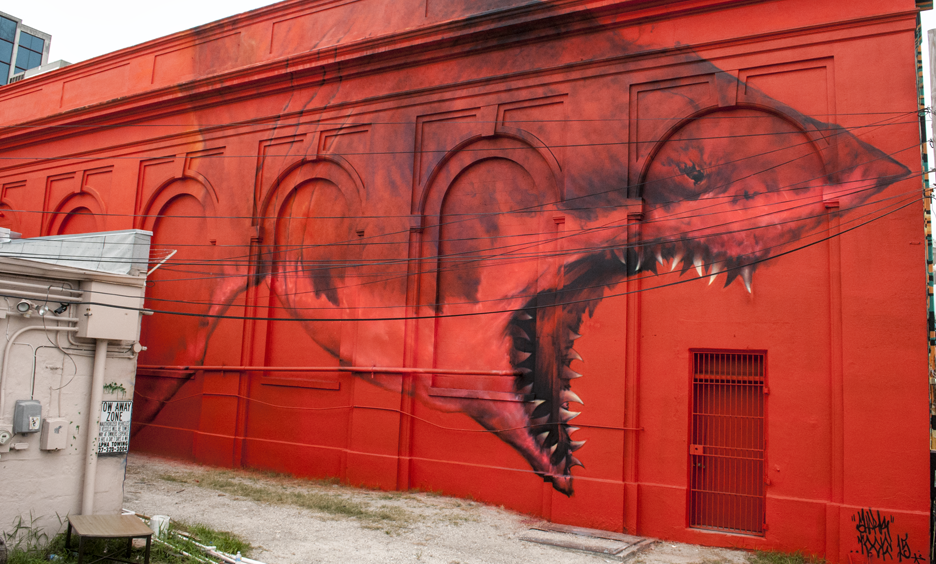The image captures a strikingly detailed mural of a menacing shark with its mouth wide open, showcasing sharp white teeth, painted on a solid red wall of what appears to be part of a stadium or a city building. The mural stretches vertically from the top to the bottom of the wall, creating a sense of depth and realism. The shark's head is depicted in vivid colors with hints of bluish black, enhancing its lifelike appearance. On the left side of the image, there is a gray power station and an electric box, with wires running across the wall. At the bottom of the photo, there is a short gray pathway. The upper left corner of the image reveals a patch of blue sky and a black object that resembles a sign. Additionally, a metal gate is present, integrated into the scene as if the shark is about to devour it. The artwork is set against a clear daytime sky, adding to the vibrancy of the entire scene.